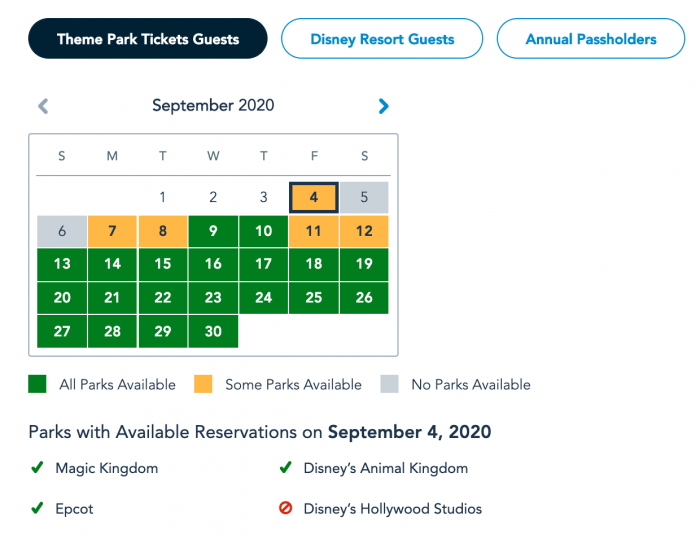The image features a user interface with a clean white background. At the top, there are three distinct buttons: the first button is black with the text "Theme Park Tickets Guests" in white; the second button to the right is white with a blue border, labeled "Disney Resort Guests"; the third button is also white with a blue border, but has a fully blue center with the text "Annual Pass Holders."

Below these buttons is a calendar interface. At the top of the calendar, there are navigation arrows: a left arrow on the left side, the text "September 2020" in the center, and a right arrow on the right side. The dates on the calendar start from Tuesday, September 1st, and end on Wednesday, September 30th.

The color-coding of the dates is as follows:
- September 1st, 2nd, and 3rd are within white boxes.
- September 4th is highlighted in yellow.
- September 5th and 6th are within gray boxes.
- September 7th and 8th are also marked in yellow.
- September 9th and 10th are green.
- September 11th and 12th revert to yellow.
- The remaining days of the month, from September 13th to 30th, are green.

A key below the calendar explains the colors: green indicates "All Parks Available," while yellow denotes "Some Parks Available."